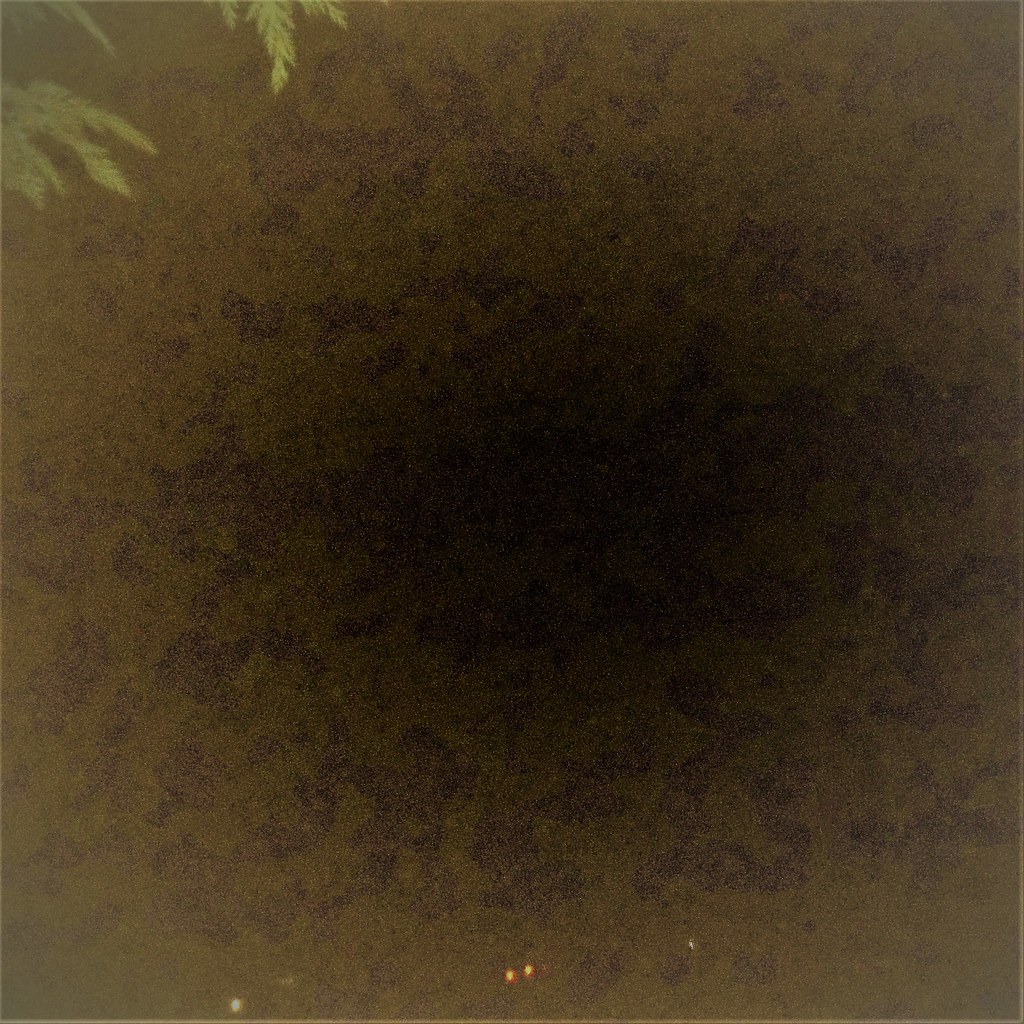This image, of very poor quality, appears to have been taken outdoors, and is predominantly dark and grainy. Most of the image is black and out-of-focus, producing a hazy and washed-out appearance. Toward the center, the blackness transitions into a greenish tint that gradually becomes lighter and more foggy around the edges. In the upper left corner, the image shows several thin leaves, likely from an evergreen tree, with three discernible branches. Additionally, near the bottom of the picture, there are a few small lights, possibly car taillights, adding a faint glow to the otherwise very dark and unclear scene.